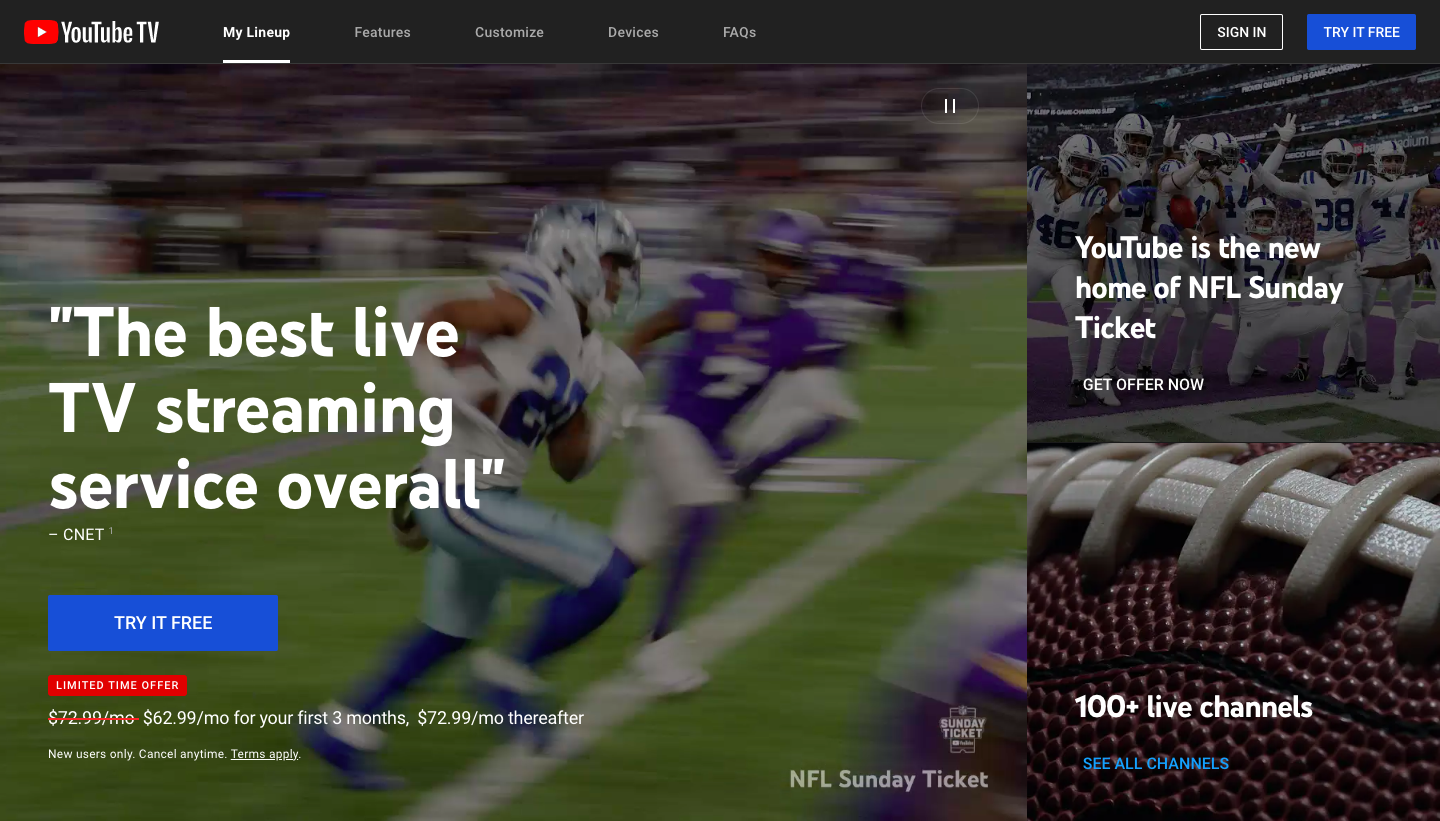This screenshot is taken from the YouTube website. At the top of the image, there is a white underline beneath the words "My Lineup." To the left, the navigation menu includes options such as "Features," "Customized Devices," and "FAQs." On the right side, there are two prominent buttons: a "Sign Up" button in white print on a black background and a "Try It For Free" button in white print on a blue background.

Scrolling down reveals an image of the Dallas Cowboys in action against a team wearing purple uniforms. Though the image is somewhat blurry, it features a large quotation overlay that reads, "The best live TV streaming service overall," attributed to CNET. Below the quote, there's another "Try It For Free" button in white print on a blue background.

A red box below the image highlights a limited-time offer: $62.99 per month for the first three months, followed by $72.99 per month thereafter. Additionally, the text emphasizes that YouTube is the new home of NFL Sunday Ticket, offering over 100 live channels.